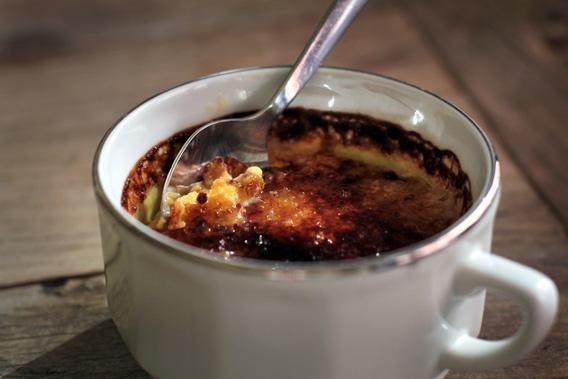The image depicts a short, stout, and wide white ceramic mug with a metallic silver edge around the top and a white handle on the right side. The mug, similar to one that would be placed on a saucer, is positioned on a wooden table characterized by mixed horizontal and vertical dark gray to brown boards with various wood striations and knotting. Within the mug, there appears to be a baked dessert, possibly a blueberry cobbler, featuring a caramelized, burnt orange, crusted top that transitions into dark purples and reds with hints of yellow. A silver spoon is partially inserted into the dessert, emphasizing its texture. The photograph is taken at a close-up angle, focusing intently on the mug and its contents.